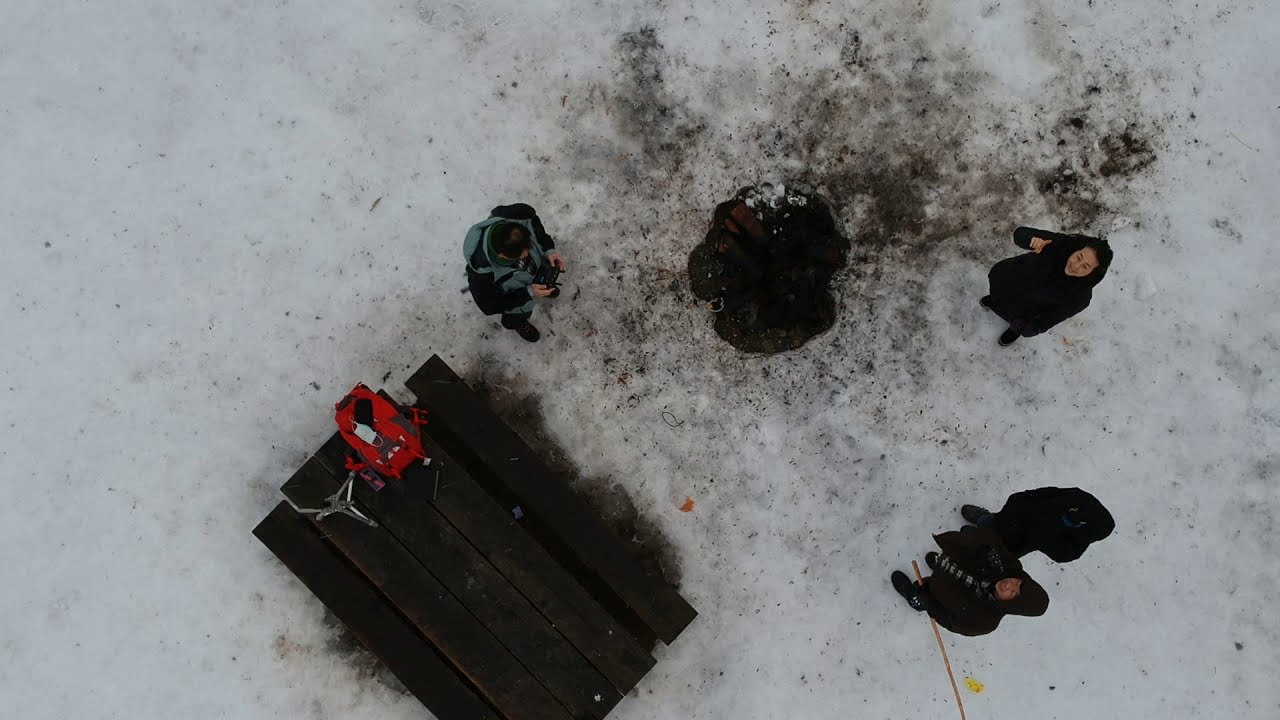This aerial image, likely captured by a drone during the daytime, shows an outdoor scene with a snow-covered ground that is partly blackened where people have been walking. The center of the image features a small group of four individuals dressed in dark, heavy coats, indicating it is a cold day. Two of them are looking up at the drone, while another is pointing upwards with her right hand, suggesting they are aware of the drone's presence. Next to the group, a dark brown picnic table holds an ambiguous red and silver piece of equipment—it could be a generator, a drone case, or another device. The area around the table and the group is dotted with possibly discarded items, and one individual appears to be holding a remote control, which might be related to the drone. The overall scene suggests a casual gathering, possibly related to ice fishing or another outdoor activity, set against a snowy and slightly muddy backdrop.